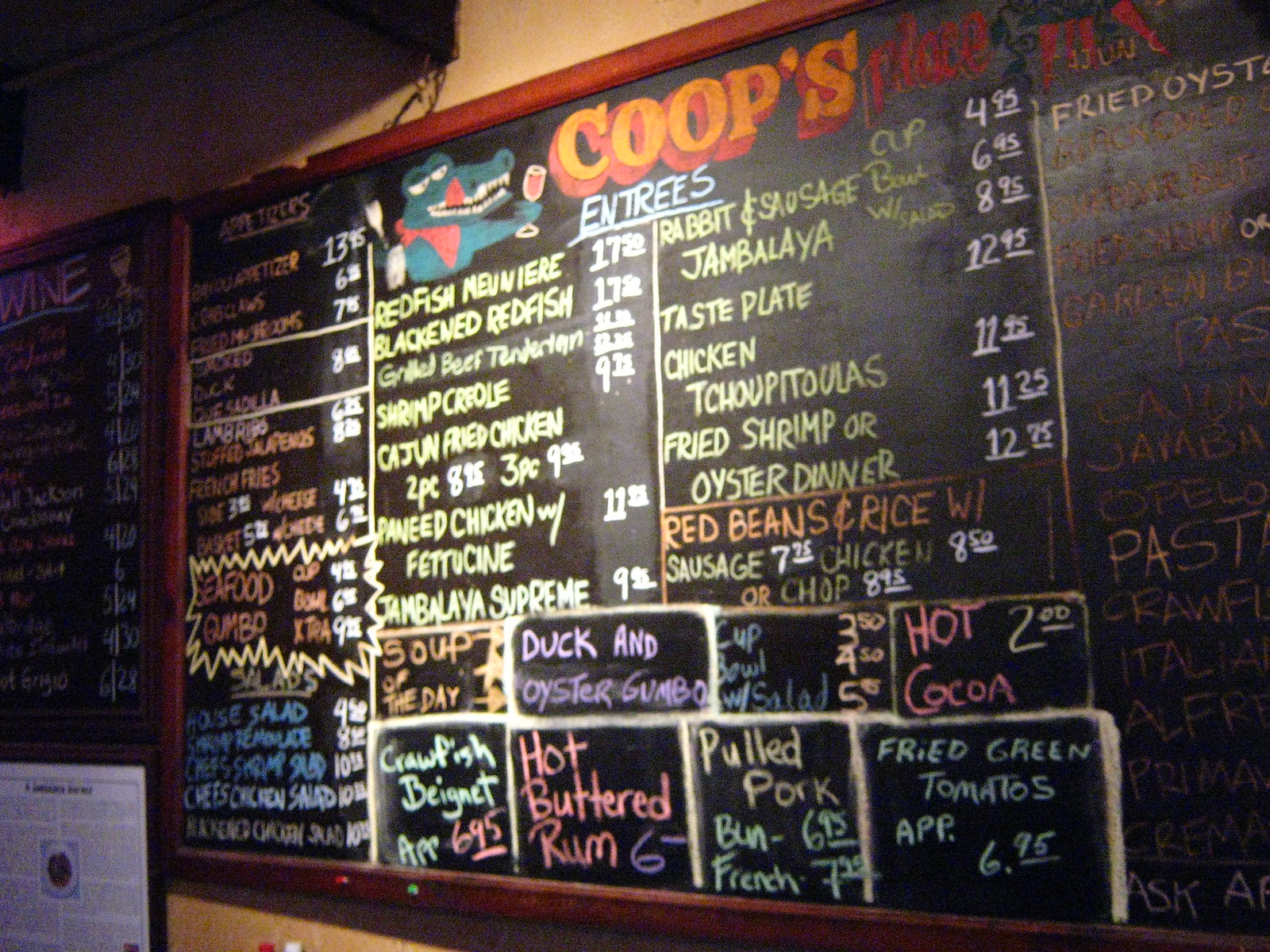This rectangular image showcases a chalk-written menu mounted on a wall, featuring two separate menu boards. The longer side of the rectangle runs horizontally. The menu on the right is partially cut off, while the left menu, set against a wooden frame, is more visibly complete. Both menus are framed with wood at the top, and the bottom of the right-hand menu is also framed.

On the upper left side of the left menu, a sign labeled "Wine" is prominently displayed, suggesting a list of wine offerings along with their prices. Below this sign is a framed article, possibly a newspaper piece about the restaurant, attached to the wall.

The primary focus of the image is the detailed right-side menu. Dominating its top section is an illustration of an anthropomorphic alligator. The alligator, depicted in green with white teeth and eyes (marked only by small dots for pupils), sports a red tongue playfully hanging out. It wears a napkin around its neck and holds a glass and a spatula, adding a whimsical touch to the menu. Beneath this illustration, the word "Koops’s" is written, followed by a comprehensive list of food and drink items available for purchase.